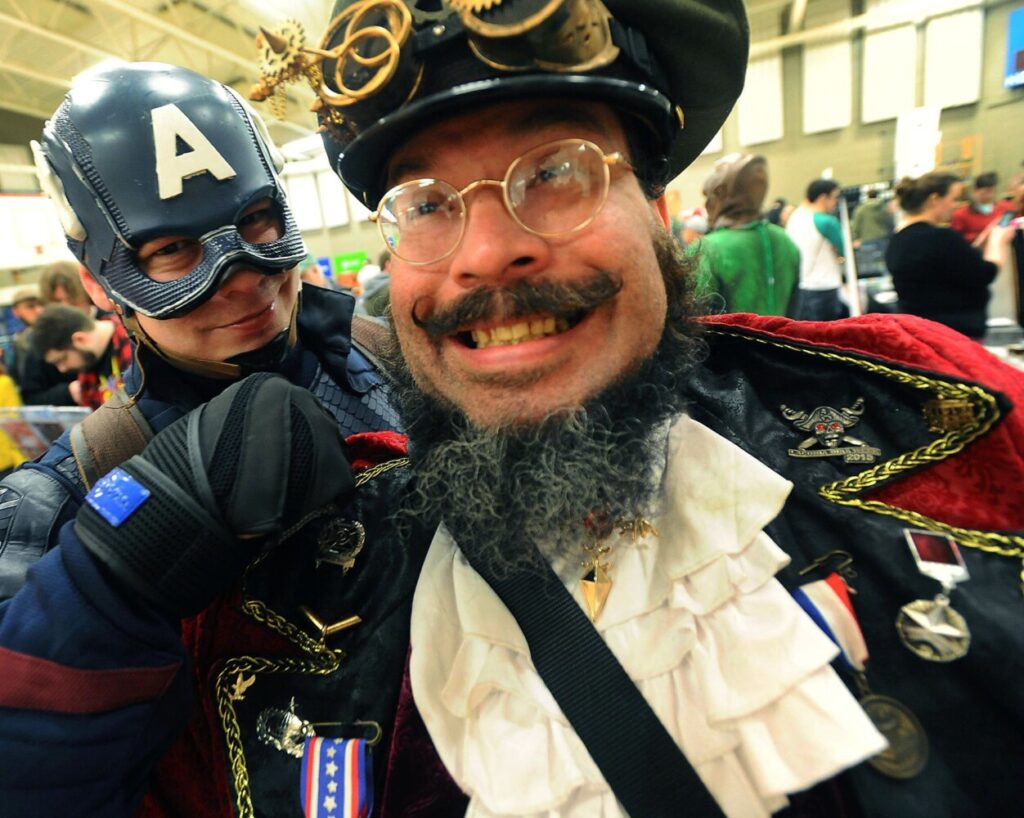This photograph, taken at a Comic-Con convention, captures the lively and engaging atmosphere of the event. At the forefront, two men are dressed in elaborate costumes, posed in a playful selfie style. To the left stands a man in an accurate Captain America costume, complete with a blue and red suit, a distinctive helmet featuring an 'A' on the forehead, and a black glove on his right hand. His right hand rests on the shoulder of his companion, who is dressed in an intricate pirate costume, accentuated by clear gold-rimmed glasses, a curling mustache, and a chin beard of curly gray hair. The pirate outfit includes a red velvet jacket with black and gold detailing on the collar, a white frilly shirt, and a black strap diagonally across his chest, possibly a bag. Adding more flair to the scene, the man taking the selfie (the pirate) sports steampunk accessories like a mechanical hat adorned with gears and goggles, and a necklace with the Ethereum symbol. Both men are smiling, exuding the cheerful spirit of the convention. In the bustling background, other attendees and various costumes add to the vibrant ambiance of the convention hall.